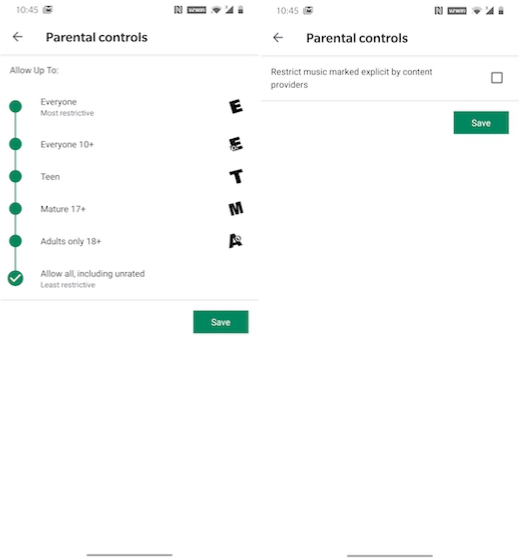This digital screenshot displays a comprehensive parental controls interface with various content rating options. At the top, the time reads 10:45. The interface includes several clearly labeled and bolded options: "Allow up to Everyone," which is the most restrictive setting. Below this setting, an uppercase bold "E" corresponds to "Everyone 10+." There is also an uppercase bold "T" for "Teen" and a bold "M" for "Mature 17+." Moreover, an "Adults Only 18+" option is denoted by an uppercase bold "A."

Each option is accompanied by a checkbox, allowing users to select or deselect content based on these ratings. On the right side, there's an option to "Restrict music marked explicit by content providers," which is currently unchecked. Additionally, there is an overarching setting labeled "Allow all, including unrated," which is the least restrictive. This setting also has a checkbox beside it. At the bottom right, a green "Save" button with white font is available to confirm and save any changes made to these settings.